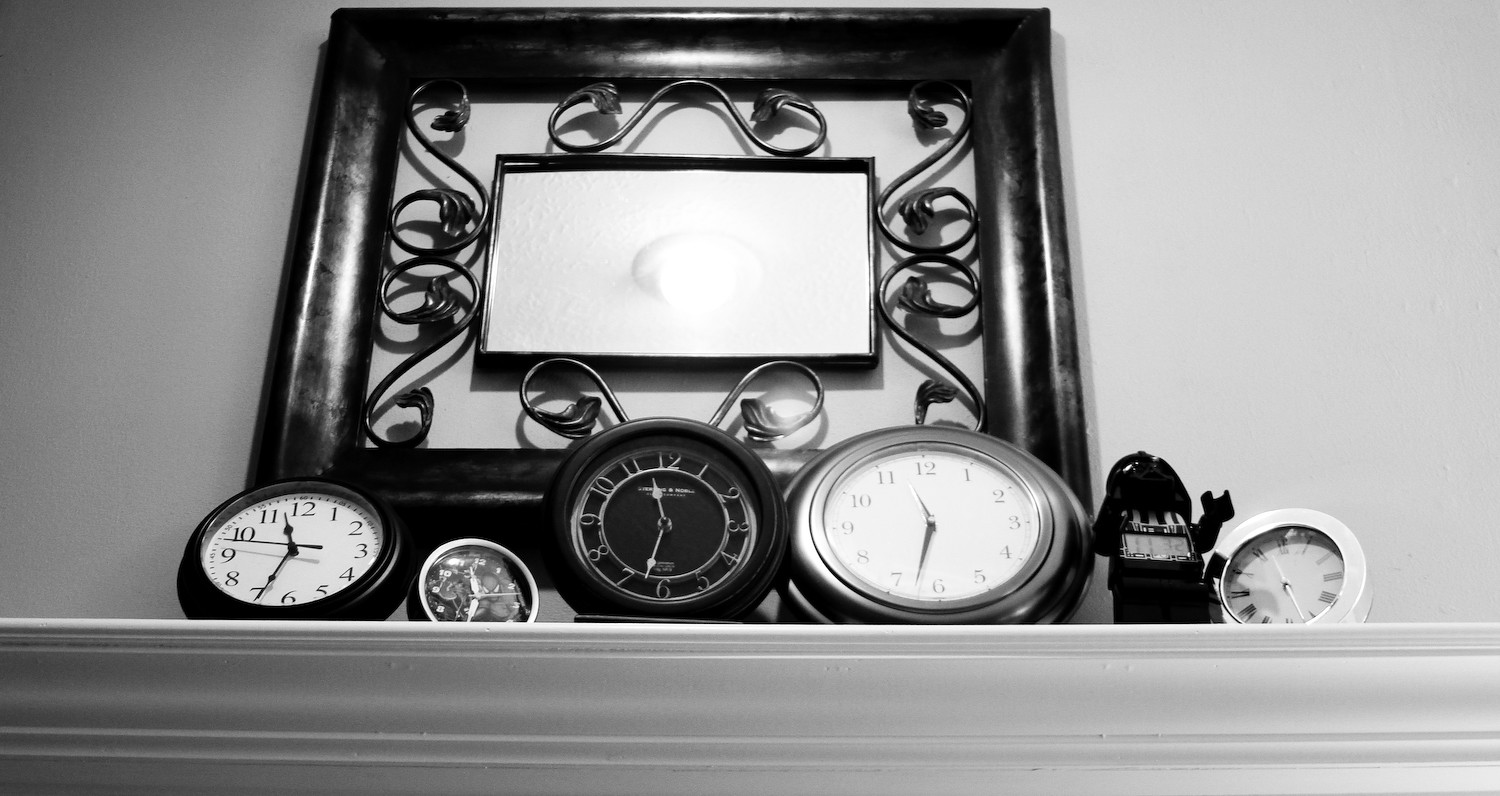This black and white photograph captures an upward view of a simple, horizontal white shelf adorned with an eclectic collection of clocks and a partially obscured, ornate framed picture. The composition includes five analog clocks, each distinguished by unique designs, and a whimsical Darth Vader digital clock, characterized by a miniature plastic Darth Vader figure with a clock embedded in his chest. Above the shelf, a square frame with intricate lattice details surrounds a smaller inset frame, though its subject remains hidden due to the intense glare. The lighting is stark and bright, casting from an angle behind the viewer, creating a dramatic and high-contrast effect that enhances the vintage and mysterious ambiance of the scene.